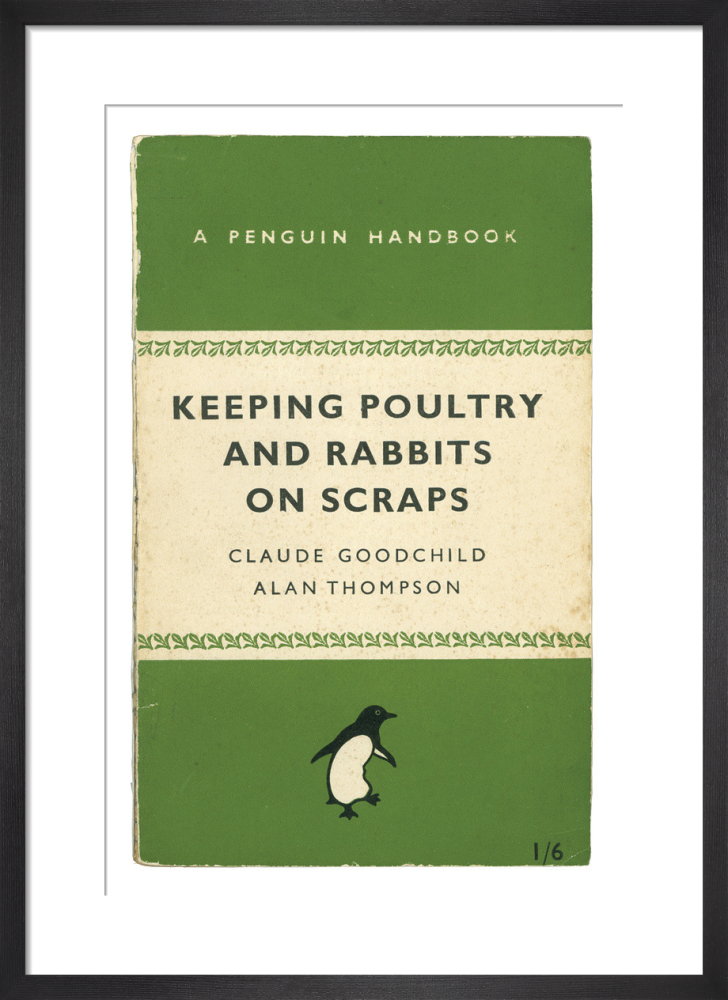The image depicts a framed cover of an older book, primarily hued in pale green with accentuating dirty off-white borders. The title section, centered in an off-white band, prominently features the book's name in black lettering: "Keeping Poultry and Rabbits on Scraps." Above this title in white letters, it states, "A Penguin Handbook." The authors, Claude Goodchild and Alan Thompson, are listed directly beneath the title. At the bottom of the cover, a black and white penguin emblem, noted for balancing on its right foot, adds a whimsical touch. In the bottom right corner, the number "1-6" could indicate that this is part of a limited print series.